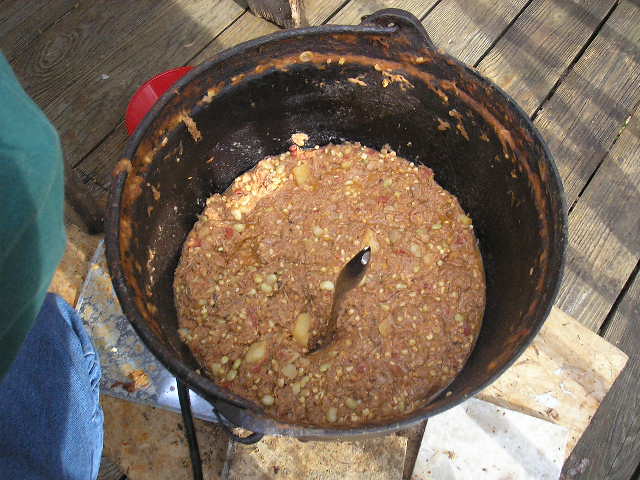The photograph, taken outdoors on a wooden deck or porch, captures a top-down view of a scene featuring a rustic cast iron pot sitting atop the wood planks. The planks themselves are old and weathered, with some square tiles strewn about, ranging in color from light tan to a single blue one. Inside the round, discolored, and slightly soiled cast iron pot is a mixture that appears to be a mash, characterized by a brown hue with occasional flecks of white and possibly chunks of potato or nuts. The pot showcases a silverware piece standing upright in the mixture. The food level in the pot appears to have dropped, indicated by a ring of residue around its rim. To the left side of the pot, a portion of a person is visible, showing just the knee of blue jeans and the shoulder of a green shirt, suggesting they might be kneeling down.